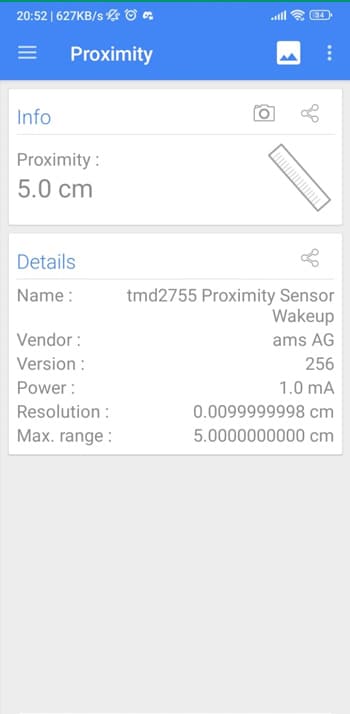This screenshot appears to be in portrait mode and is formatted as a long column. The background has a light blue section with a green stripe in the upper left corner.

At the top left corner, there’s the number "2052," and at the top right corner, a battery icon shows "34%." Directly below these, there are three horizontal lines stacked on top of each other, followed by the word "Proximity" and an image icon.

The next row, with a white background and blue text, has the word "Info" on the right side, next to icons for a camera and sharing.

In the subsequent row, it reads "Proximity 5.0 centimeters" accompanied by a ruler icon.

Another block of content follows, also with a white background and blue text, showing "Details" on the left and "Share" on the right.

Further down, it lists specifics including: 
- "Name: TMD 2755 Proximity Sensor Wake Up"
- "Vendor: AMS AG"
- "Version: 256"
- "Power: 1.0 mA"

The text then details the sensor's resolution, listed as "0.0099999998 centimeters," and its maximum range of "5 centimeters."

The proximity sensor data, indicating a range of just five centimeters, suggests a very close measurement capability, which might be used for detecting objects within half an inch of the sensor's surface. This detailed information potentially relates to a monitoring or detection function.